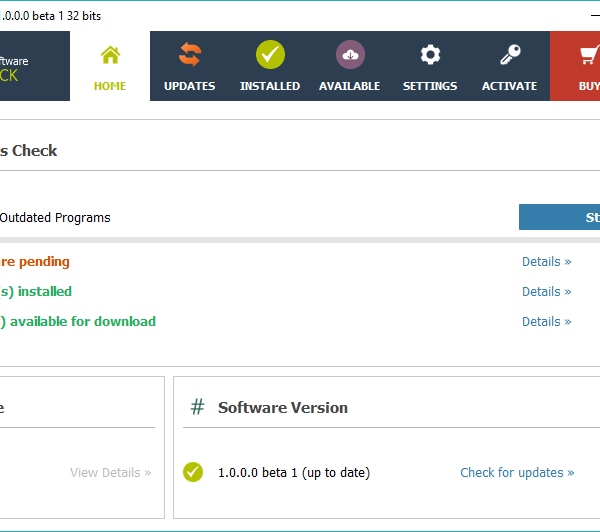A screenshot displays the top portion of an antivirus or anti-malware application. The toolbar includes several tabs labeled Home, Updates, Installed, Available, Settings, Activate, Buy, and Outdated Programs. The statuses indicate that some updates are pending, some programs are installed, and others are available for installation. The application version is shown as "Software Version 1.0.0.0 Beta 1." A green check mark indicates that the software is up-to-date, with an option to "Check for Updates." The screenshot provides a detailed overview of the software's current status and available actions.